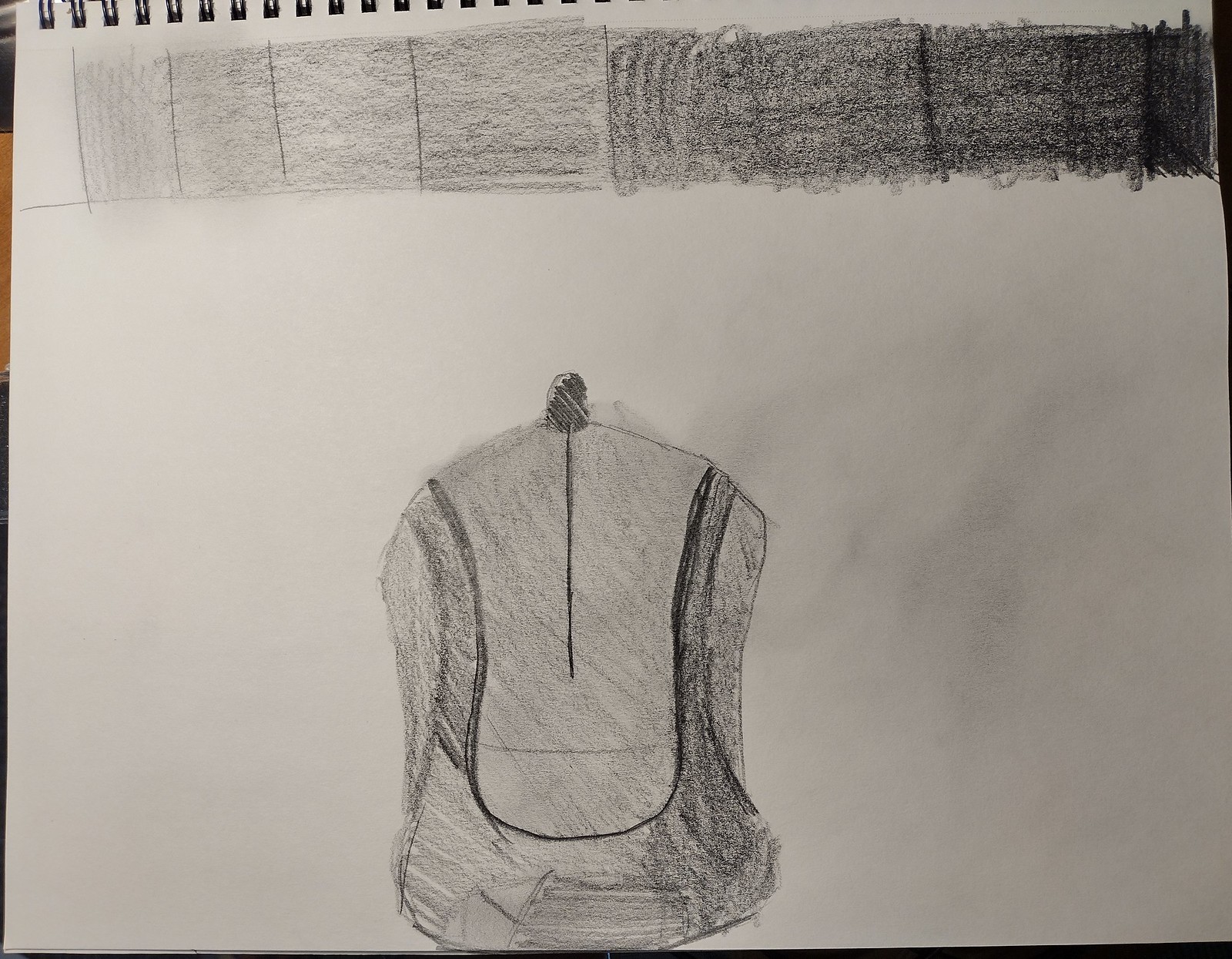This black and white pencil sketch, drawn on a spiral-bound sketchpad, depicts a detailed combination of geometric shapes and a piece of clothing. At the top of the drawing are a series of squares and rectangles, arranged side by side, with visible lines in between. These shapes are shaded in varying intensities; the boxes on the right are filled darkly with pencil, transitioning to lighter shades towards the left, eventually leaving the leftmost box uncolored. This gradual change in shading creates a sense of depth and dimension. Below this geometric pattern, the illustration features an ambiguous piece of clothing, possibly a jacket or a vest. This garment, detailed with a line down the middle and long sleeves, has darker shading on the right side and lighter shading on the left, suggesting light sourcing. Additional features, such as potential straps or outlines around the chest area, add to its complexity. The overall image is rich in shading details, contributing to a textured, layered look that brings both the geometric forms and the garment to life.